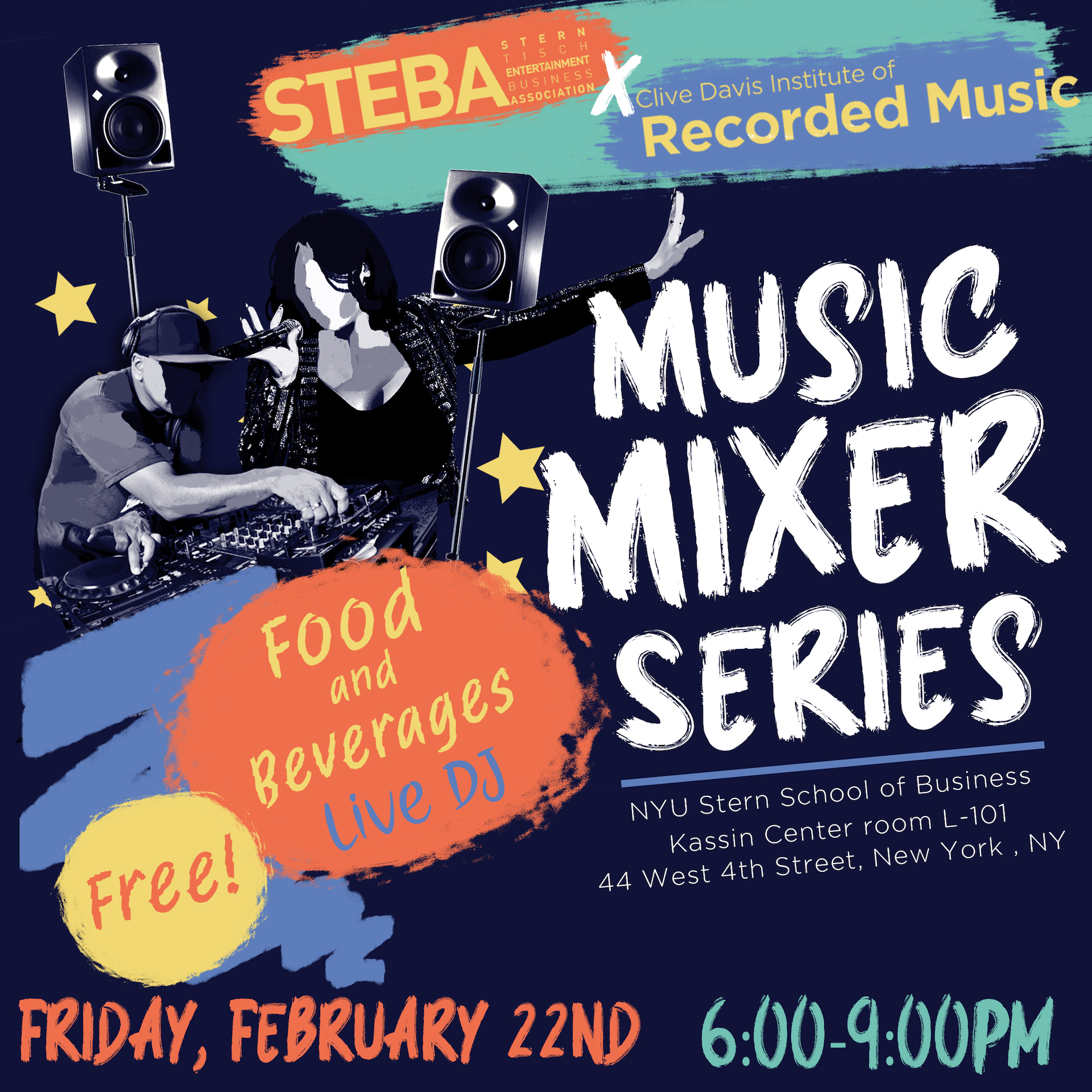Promotional Poster Description:

This eye-catching promotional poster advertises the "Music Mixer Series" concert, an event organized by the Stebba Stern Entertainment Business Association in collaboration with the Clive Davis Institute of Recorded Music. The design features a prominent image of a DJ and a woman holding a microphone, both illustrated in a grayscale style with shaded-out faces, giving them a computerized, abstract look. The DJ is shown with a mixing keyboard, enhancing the musical ambiance of the poster.

Key event details are vibrantly highlighted in contrasting colors. "Friday, February 22nd" is written in a bright orange, while "6 to 9 p.m." is displayed in an aquamarine blue-green hue. Additional text indicates that there will be food, beverages, and a live DJ, making it clear that attendees can expect a lively and entertaining evening.

The event's location is specified as the NYU Stern School of Business, Cassin Center room L101, situated at 44 West 4th Street, New York, New York. The Clive Davis Institute's name appears with an artistic flair, mimicking an ink paint smear, contributing to a street-art aesthetic. The background features a dark blue, almost black hue, creating a striking contrast with the highlighted text and making the details pop.

Overall, the poster combines modern digital art with vibrant colors and detailed event information, making it an engaging and informative advertisement for the event.